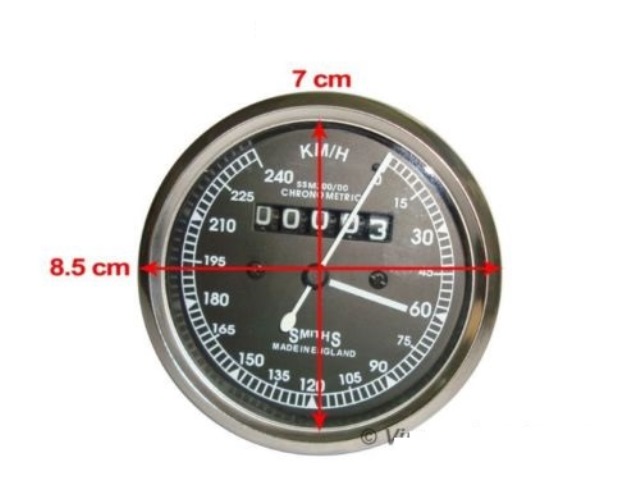This image features a vintage analog speedometer, which measures speed in kilometers per hour (km/h). It does not use the American miles per hour (mph) system. The speedometer has a distinctive design with a silver outer ring and a black central circle, which is marked with white indicator lines and numbers. The numerical markings are in increments of 15, starting from 0 and going up to 240. The text on the speedometer includes the term "chronometric," which may refer to its precision mechanism, and there are additional numbers likely indicating brand identification.

The odometer displays only 3 kilometers, but the dial appears capable of recording up to 99,999 kilometers. Manufactured by Smith's, the device is marked "Made in England." Given its analog nature and potential age, it suggests that this speedometer might be from a classic or older model car, as modern vehicles often utilize digital speedometers.

The dimensions of the speedometer are prominently noted as being 7 centimeters in length and 8.5 centimeters in width, suggesting that these details are important, possibly for purposes of sale. This detailed caption provides an in-depth look at the item, likely aimed at prospective buyers or collectors seeking vintage automotive instruments.